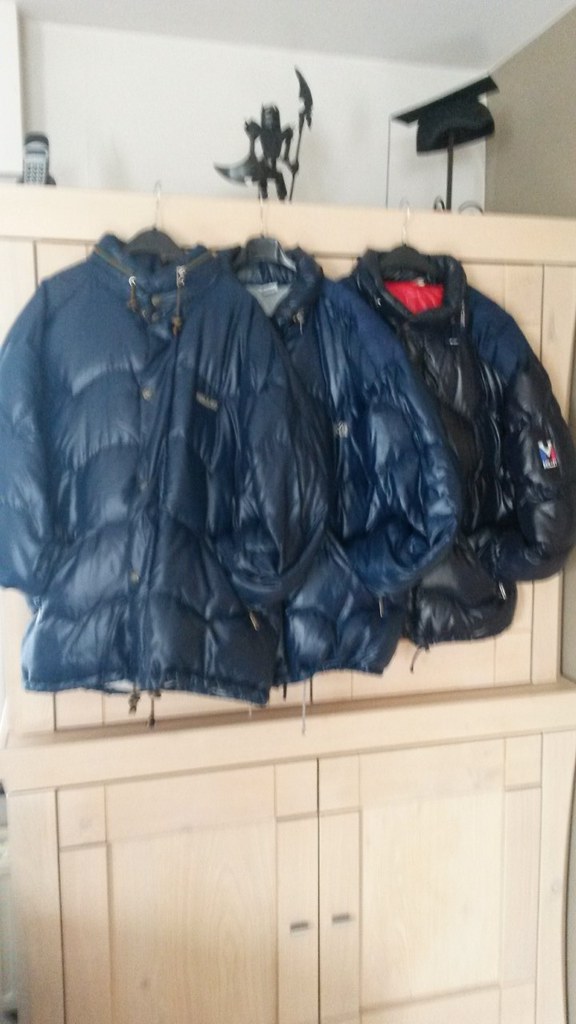This indoor color photograph depicts three puffy blue winter jackets, likely skiing jackets, hanging on brown hangers with steel hooks from a light maple dresser or chest of drawers, which spans the entire height of the image. The jackets, all fully zipped, are positioned in the upper half of the frame. The leftmost jacket is a medium blue, while the middle one is slightly darker, and the rightmost jacket is the darkest blue with a visible red lining at the neck. The jackets feature drawstrings around the neck and bubble-like puffs throughout their fabric. The dresser has a natural wood finish, adorned with silver handles. Atop the dresser, there's a metal statue or figurine of a creature wielding a large axe and wearing a bucket helmet, flanked by an old-style gray cell phone to the left and a graduation cap to the right. The background includes a white wall directly behind the cabinet and a tan-colored wall to the right, providing a well-lit, though slightly out-of-focus, backdrop for the scene.